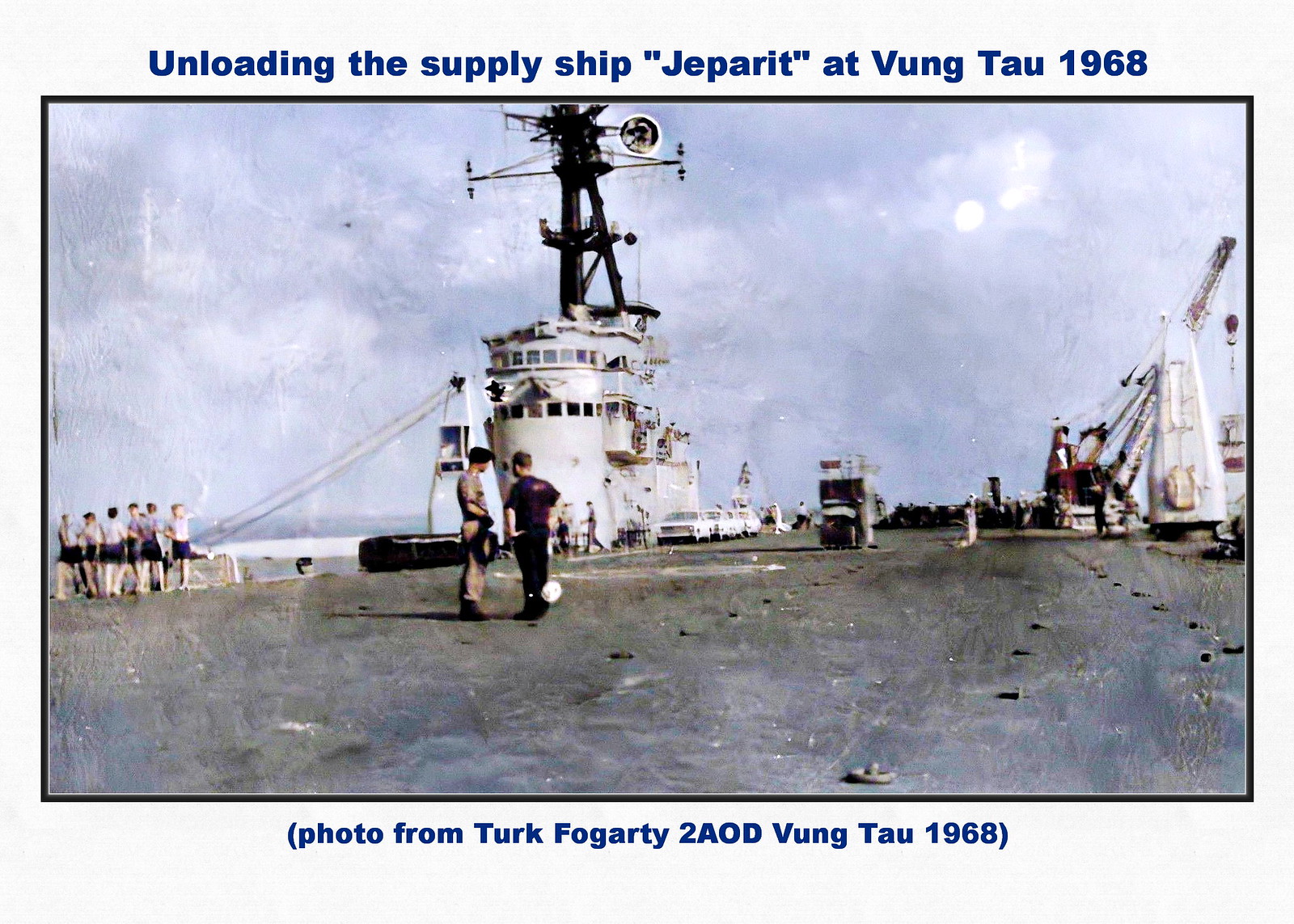The photo, titled "Unloading the Supply Ship Jeparit at Vung Tau 1968," is from Turk Fogarty to 2AOD Vung Tau 1968. It captures a moment in 1968 Vietnam, portraying a horizontally oriented 16x9 landscape image of the top of a large supply ship named Jeparit. The ship, featuring a tall mast with sonar equipment at its apex, is framed against a backdrop of overcast gray clouds with a bright hotspot in the upper right. On the right side of the image, an oil rig or crane is visible, adding industrial context to the scene.

In the central portion of the image, a small group of individuals, likely young men or teenagers dressed in black shorts and light gray tops, can be seen gathered at the edge. In front of the tall ship, there are two distinct figures. On the right, one person is clad in dark clothing, while the person on the left wears khaki attire along with a hat. The person in khaki is possibly in a uniform, suggesting a more official role. The overall ambiance is predominantly gray, highlighting the metallic surface of the ship and the cloudy sky, which contributes to a somber, stationary feel with no evident motion or blurriness in the image.